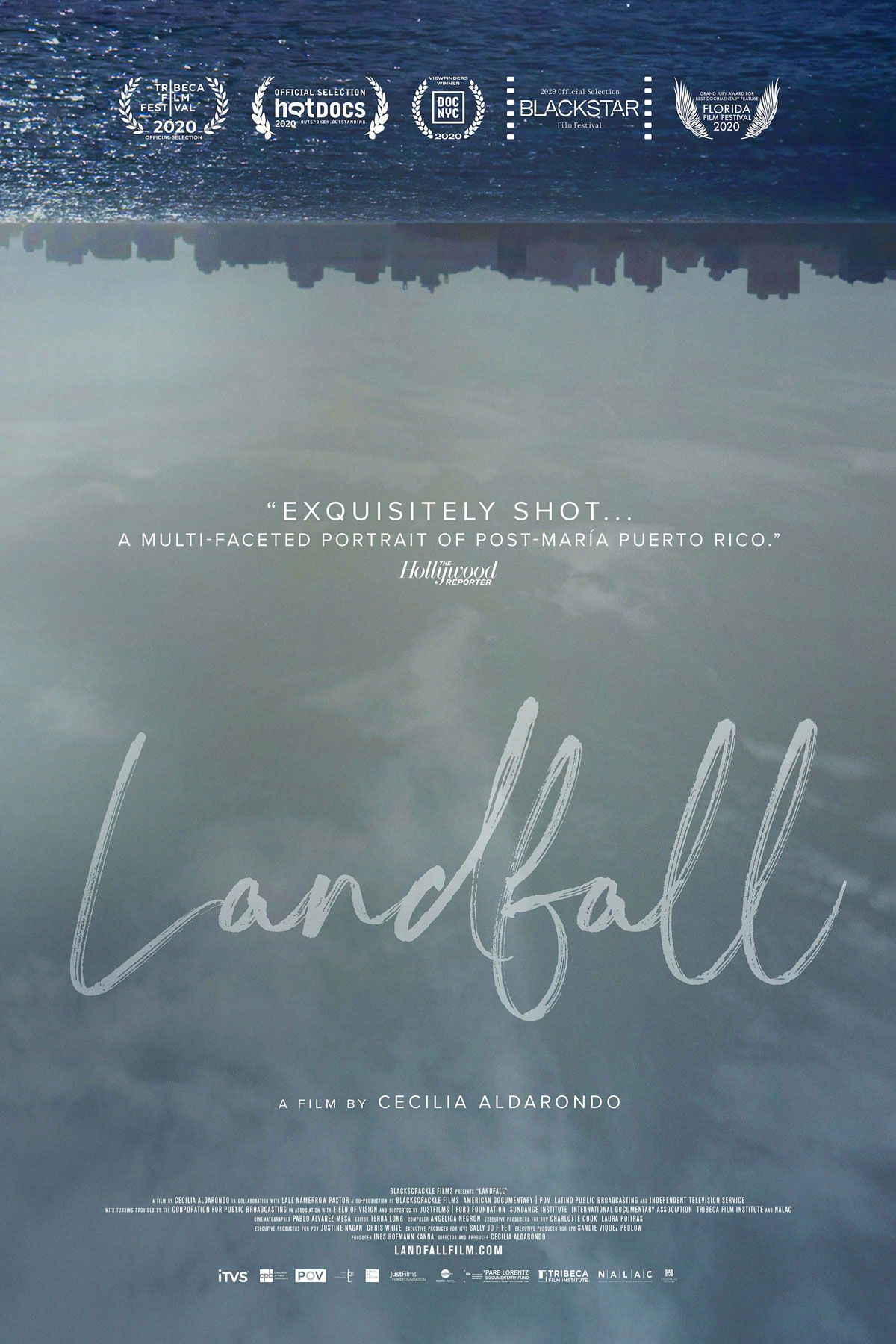This is a highly detailed movie poster for "Landfall," a film by Cecilia Aldarondo. Dominated by blue and gray tones, the poster features an evocative, inverted landscape. At the top, we see a cityscape above a rocky shoreline with water beneath. The water's surface reflects the skyline above, creating a striking visual of an upside-down city. At the very top of the image, various festival accolades are displayed, including Tribeca Film Festival 2020, Official Selection Hot Docs 2020, DOC NYC 2020, Black Star Film Festival 2020, and Florida Film Festival 2020.

Centered in the poster is the quote "exquisitely shot, a multifaceted portrait of Post Maria, Puerto Rico," credited to The Hollywood Reporter. Below the quote, the movie title "Landfall" appears in elegant cursive, followed by "a film by Cecilia Aldarondo." Additional information at the bottom mentions ITVS, Tribeca Film Institute, Black Crackle Films, and the movie's website, Landfall.com. The overall composition artfully captures the essence of the film, enticing potential viewers with its aesthetic and critical acclaim.